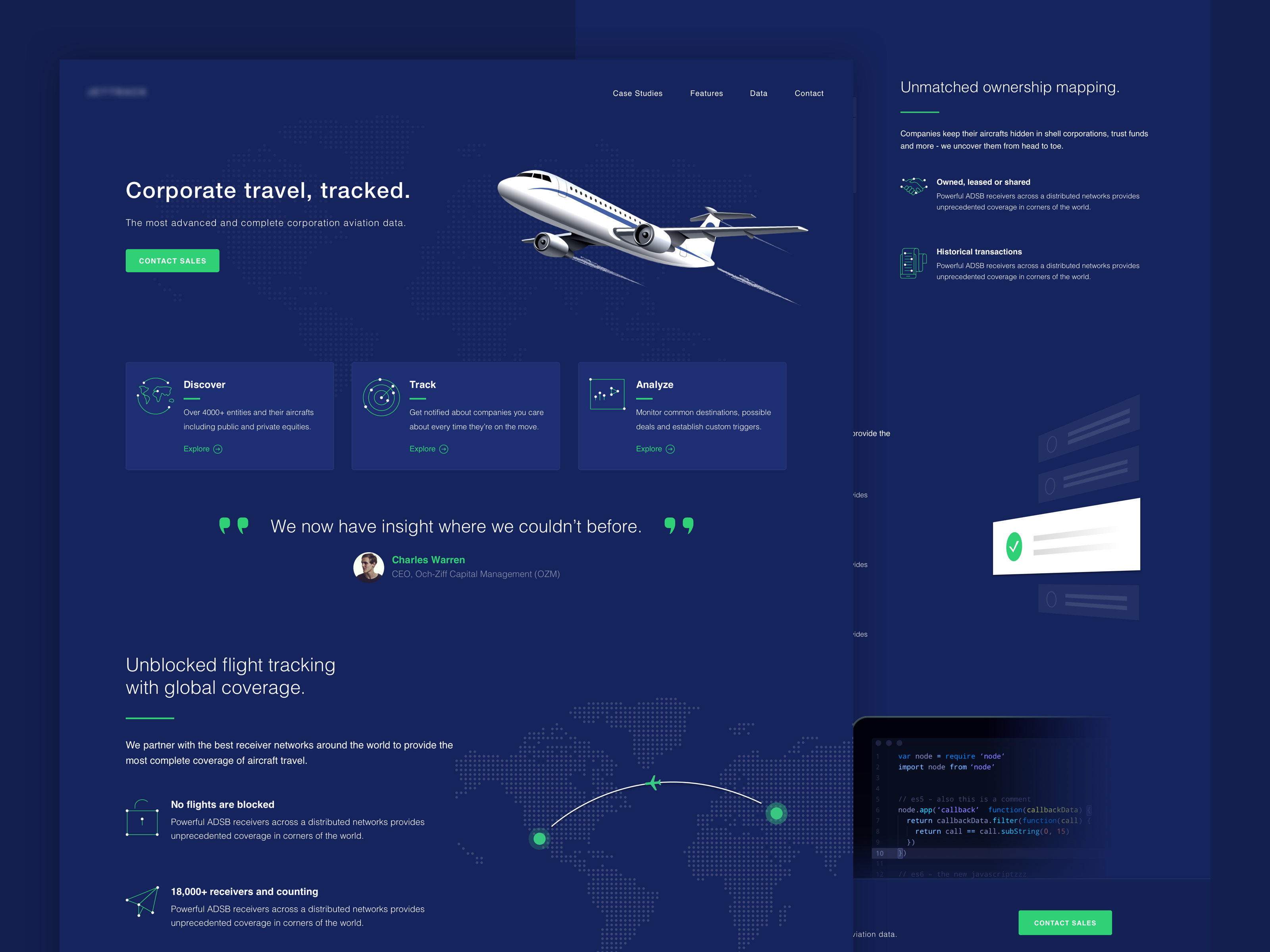The screenshot showcases a travel website tailored for corporate aviation, featuring a sleek, purplish-blue theme with a dark hue. Dominating the top part of the page is an image of a passenger plane ascending towards the top-left corner. Adjacent to the image, a bold title reads "Corporate Travel Tracked the Most," followed by a subtitle in smaller white text stating, "The most advanced and complete corporate aviation data." Below this header, a prominent green "Contact Sales" button invites user engagement.

Three interactive boxes are aligned horizontally below the main section. The first box, labeled "Discover," is followed by "Track" in the second box and "Analyze" in the third. Beneath these boxes, there is a quote prominently displayed in white text nestled within green quotation marks. The quote, given by Chris Warren, the CEO of a company, reads, "We now have insight where we couldn't before."

At the bottom of the web page, a detailed map of the world appears, depicted in a flat layout with continents illustrated by tiny blue dots. Southern California is marked by a large green dot, connected by a curved white flight path that spans across the Atlantic Ocean to another green dot in Turkey. 

To the left of the map, a heading declares "Unblocked Flight Tracking with Global Coverage." Below the heading are two constellation-style icons. The first icon resembles a lock and is accompanied by the text "No flights are blocked," while the second icon, depicting a paper plane, indicates "18,000+ carriers and counting."